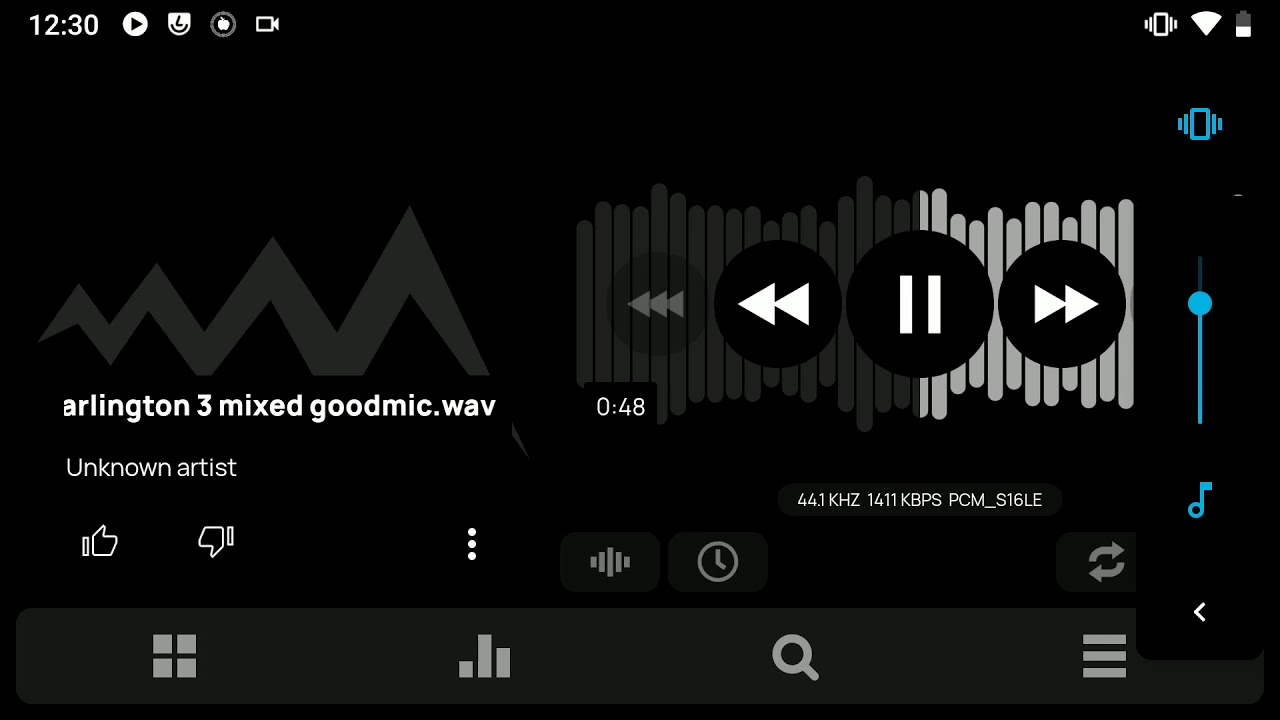The image appears to be a screenshot of a music streaming platform's interface. At the top, the background is solid black with white text and gray graphics, accented by sky blue elements. On the left, a status bar displays the time, "12:30." Following this, there are icons for play, an Apple device, and a camera. Toward the right side of the status bar, you can see WiFi and battery icons.

Directly below, a sky blue bar, likely indicating volume control, and a sky blue musical note are visible. To the left of this bar are playback controls, including a fast forward button, a pause button, and a reverse button. Behind these elements, vertical lines in dark gray and light gray create a textured background. A timestamp beneath these controls reads "04:48."

Further down, there's a zigzag line, possibly an audio waveform, with the text "Arlington 3 mixed good mic dot way" underneath. Below this text, "Unknown Artist" is displayed. Next to the artist's name, there are thumbs up and thumbs down icons for rating the track. To the right of these icons are three vertical dots indicating additional options. Adjacent to this, there is an unfamiliar icon composed of five horizontal lines.

To the right of the five-line icon, there is a clock icon, followed by a repeat icon showing two curved arrows stacked one above the other. At the bottom of the interface, four icons are presented: a grid icon consisting of four gray blocks, vertical bars of varying height, a search icon, and a hamburger menu icon.